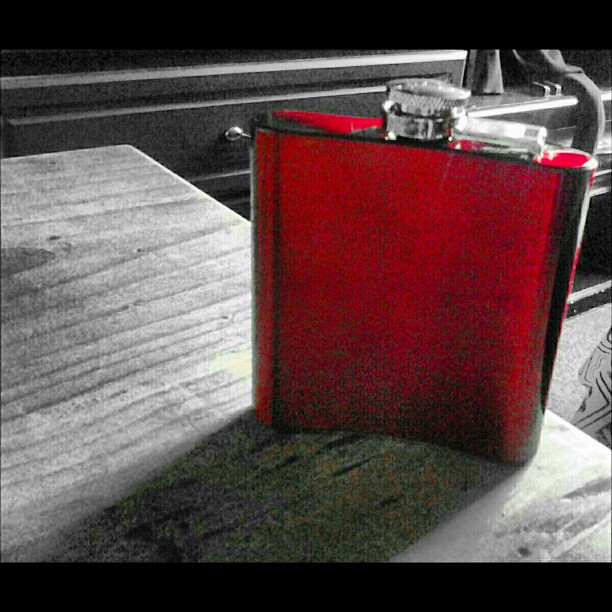A beautifully artistic photograph features a striking juxtaposition of colors and textures. Rendered predominantly in black and white, the central focus of this close-up image is a red metallic flask with a silver screw top, meticulously colorized in post-processing to stand out against its monochrome surroundings. The flask, with its curved portion facing towards the viewer and black accents highlighting its contours, casts a shadow onto the wooden table it rests upon. The table, seemingly part of a cozy apartment setting, is joined by a hint of a cabinet handle and a possible carpet visible in the blurred black and white background. The flask appears small and handheld, typical of stainless steel designs, and the light reflecting off its silver top adds a dynamic element to the composition. The photograph is framed with a black header and footer, enhancing its artistic presentation and ensuring that all attention is drawn to the vivid red flask that commands the viewer's gaze in this otherwise serene and timeless scene.